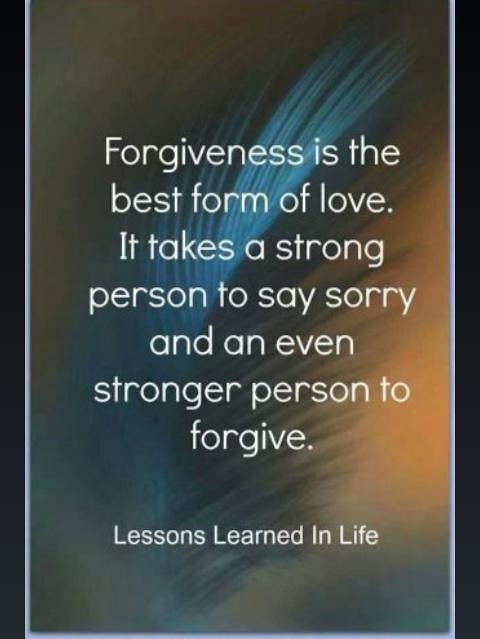This image depicts an inspirational card with a dark grayish background accented by streaks of light blue and burnt orange. It features black borders on the left and right sides, and shows a clean, white font that delivers a powerful message: "Forgiveness is the best form of love. It takes a strong person to say sorry and an even stronger person to forgive." The card, possibly part of a series titled "Lessons Learned in Life," emphasizes the importance of forgiveness as a vital life lesson. The backdrop, shadowy and streaked with subtle colors, enhances the card's profound message.